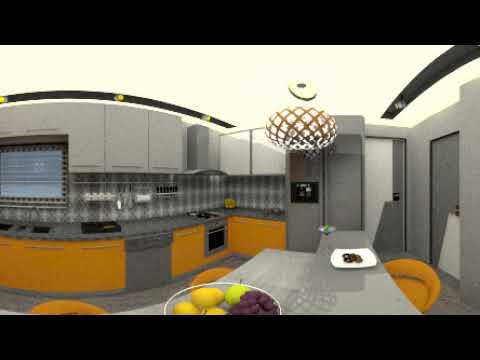The image depicts a spacious, modern kitchen with a predominantly gray and orange color palette. The dazzlingly white ceiling features black inlet tiles and a unique light fixture with brown bands. The upper cabinets are a sleek gray, while the bottom cabinets and a few surrounding chairs are a striking orange, providing a bold contrast. Central to the image is a large, curved table with what looks like a gray granite surface. On the table, there is a transparent bowl with a stainless steel rim containing grapes, pears, oranges, and a mango. Adjacent to that bowl is a white tray that might hold cookies.

The kitchen includes a small stainless steel refrigerator, a small stove with an oven, and a black sink situated in front of a large window that allows ample natural light. The countertop, appearing to be made of a gray plasticky material, has a white and gray tile backsplash. There's also a towel rack and additional storage options like a pantry door, a hallway door, and potentially another door leading out of the kitchen. The ambiance is high-tech, accentuated by small lights above the cabinets and reflective surfaces that add depth to the space.